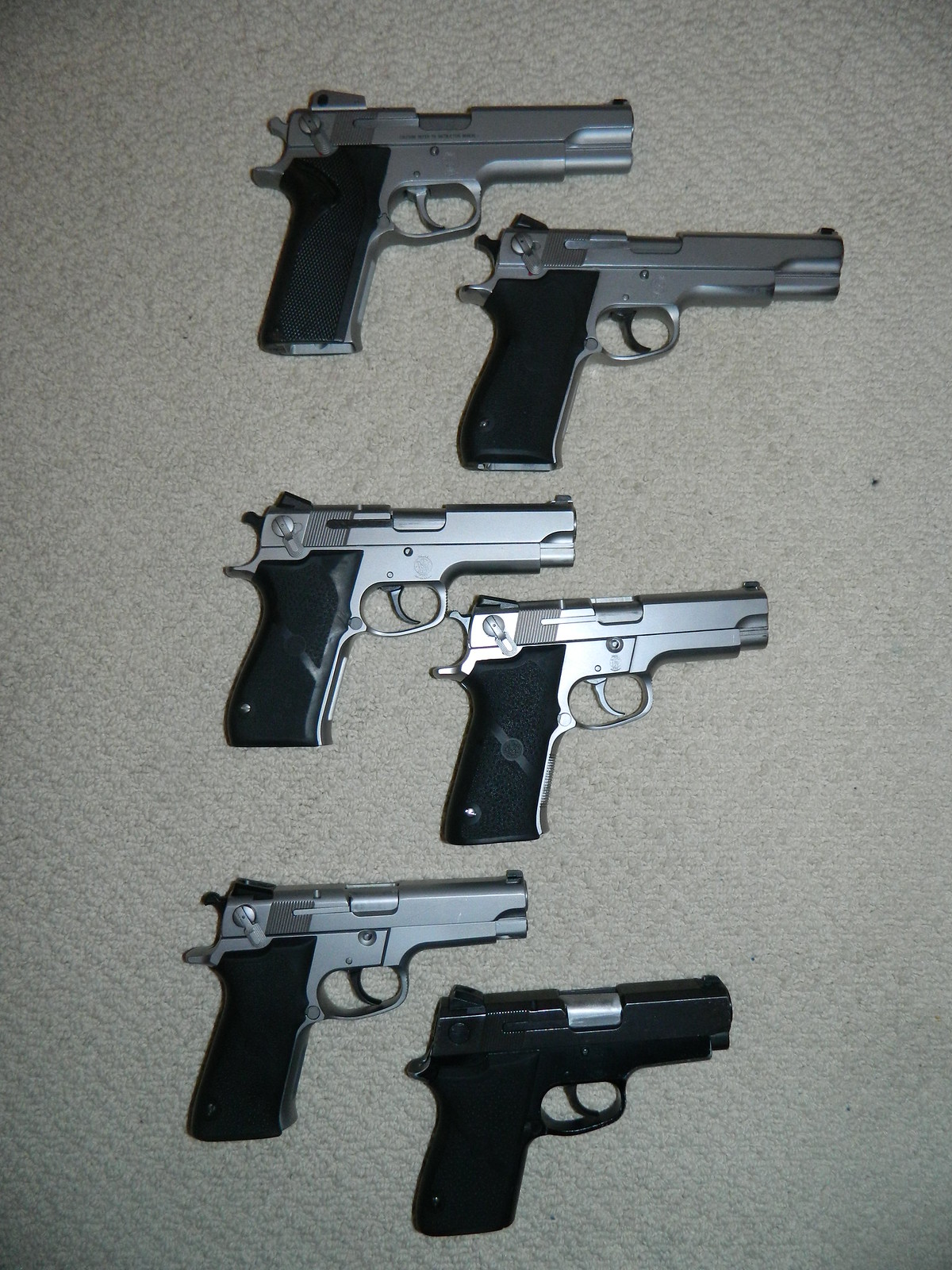The image depicts six handguns meticulously arranged on what appears to be a beige, Berber carpet. Five of the handguns feature a shiny, metallic silver body paired with black composite plastic handles, indicating they are fairly new and unused. The sixth handgun stands out with its predominantly black metal body, complemented by a small stainless steel section on top. Each firearm is oriented with the barrel pointing to the right and the handles on the left. Notably, the triggers of two of the silver handguns are black, while the remaining three have silver triggers. The black handgun also has a matching black trigger. All the firearms are organized in three pairs: two at the top, two in the middle, and two at the bottom, presenting a uniform and orderly arrangement.